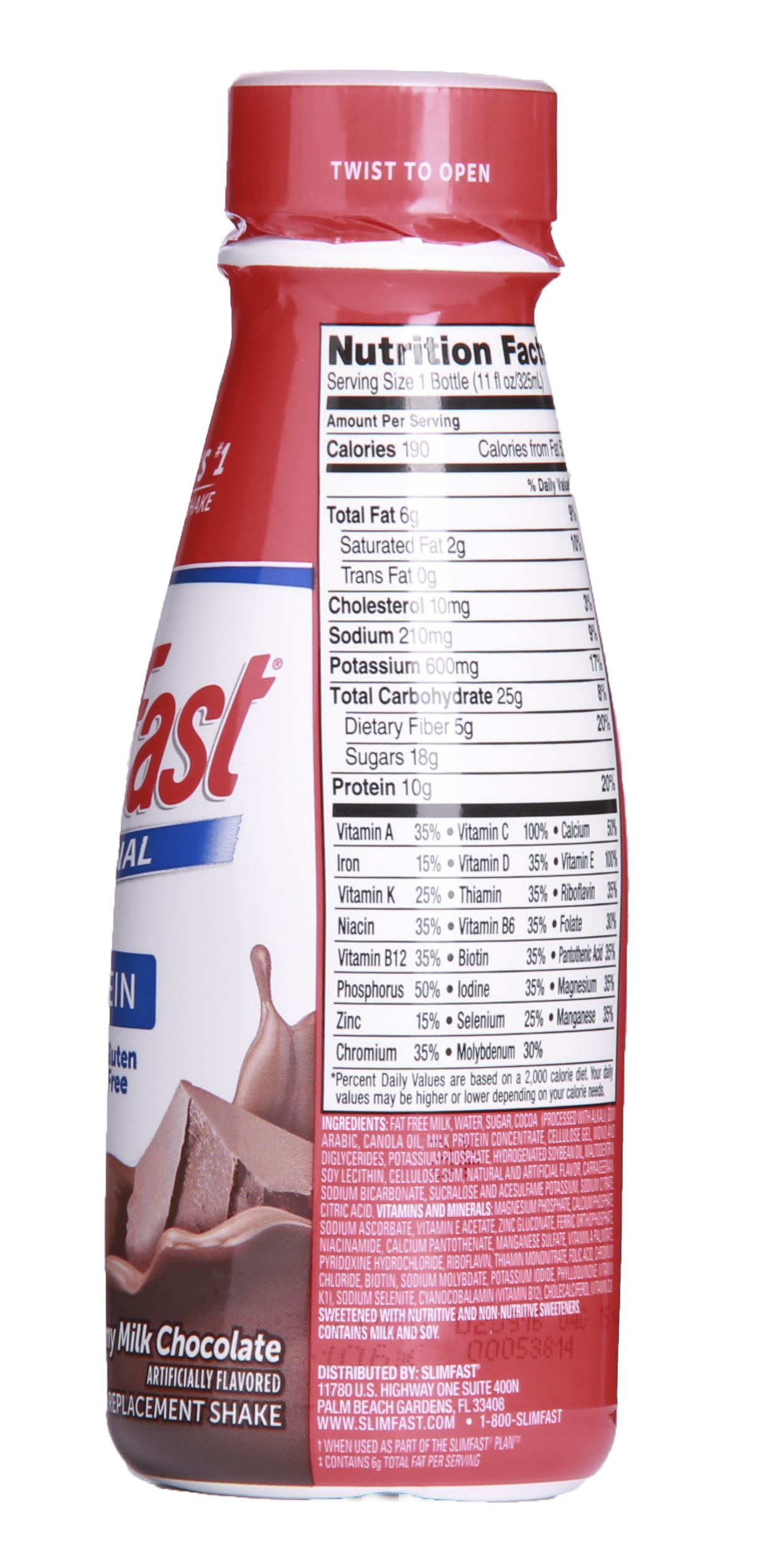This is a detailed photograph of an 11-fluid ounce SlimFast weight loss drink with a milk chocolate flavor. The bottle, predominantly red, lies on its side against a plain white background, displaying the side profile of its label. The visible portion of the label shows the partial brand name "AST" and features a blue line under it. At the bottom of the label, there's an illustration of chocolate pieces and the word "chocolate" written in white. The back of the bottle, which is white, displays the nutritional facts in black text. The drink provides 190 calories, 2 grams of fat, 10 milligrams of cholesterol, 210 milligrams of sodium, 600 milligrams of potassium, 25 grams of carbohydrates, 5 grams of fiber, 18 grams of sugar, and 10 grams of protein. Additionally, the label lists various vitamins and minerals, including vitamins A, K, B12, C, D, B6, zinc, biotin, and iodine, along with other detailed percentages. The bottle also mentions the official website at the bottom: www.slimfast.com.